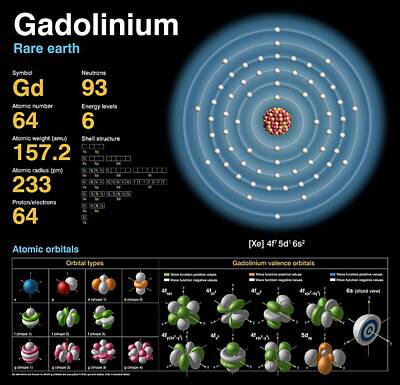This detailed black poster prominently showcases scientific imagery and information. In the upper left corner, the word "Gadolinium" is displayed in bold white letters, while "Rare Earth" is written in striking blue letters. To the right, a large multi-layered circle dominates the design. At its core, numerous small dots in shades of purple, brown, and white are clustered together. Surrounding this central area, the circle consists of various layers in different hues of blue, each adorned with tiny white dots, creating a concentric pattern.

At the bottom of the poster, a chemical formula, "XC4F5D6S," is neatly printed, suggesting a complex molecular structure. Below this, images of different molecules are arranged, accompanied by the label "Atomic Orbitals." Numerous numbers and details are interspersed throughout, adding depth and scientific context to this visually arresting and informative poster.